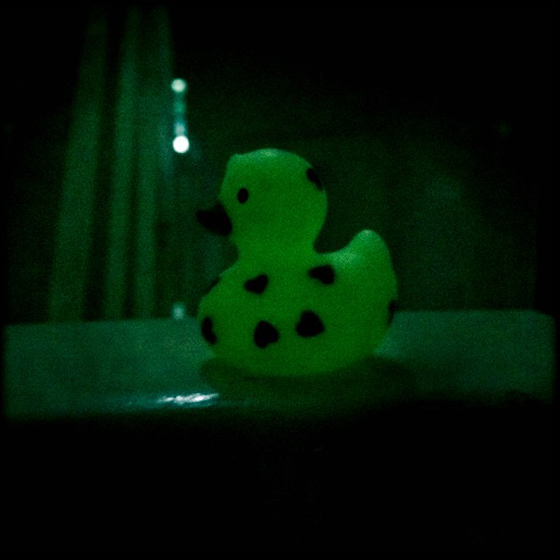The image is a dimly lit photograph capturing a small plastic toy duckling, likely rubber, which appears to be green with numerous black heart-shaped dots scattered across its body. The room is nearly dark, likely illuminated by a single weak light source, providing just enough light to outline objects. The duck, facing left with its small black beak and eyes, sits on a smooth, reflective surface that could be a countertop, showing spots of bright white shine. Behind the duck, the background includes ripple-textured curtains that are faintly visible due to their placement on the wall and the reflection of the minimal light. The overall scene has a very dark ambiance, giving the toy duck a subtle neon glow effect against the shadowy surroundings.